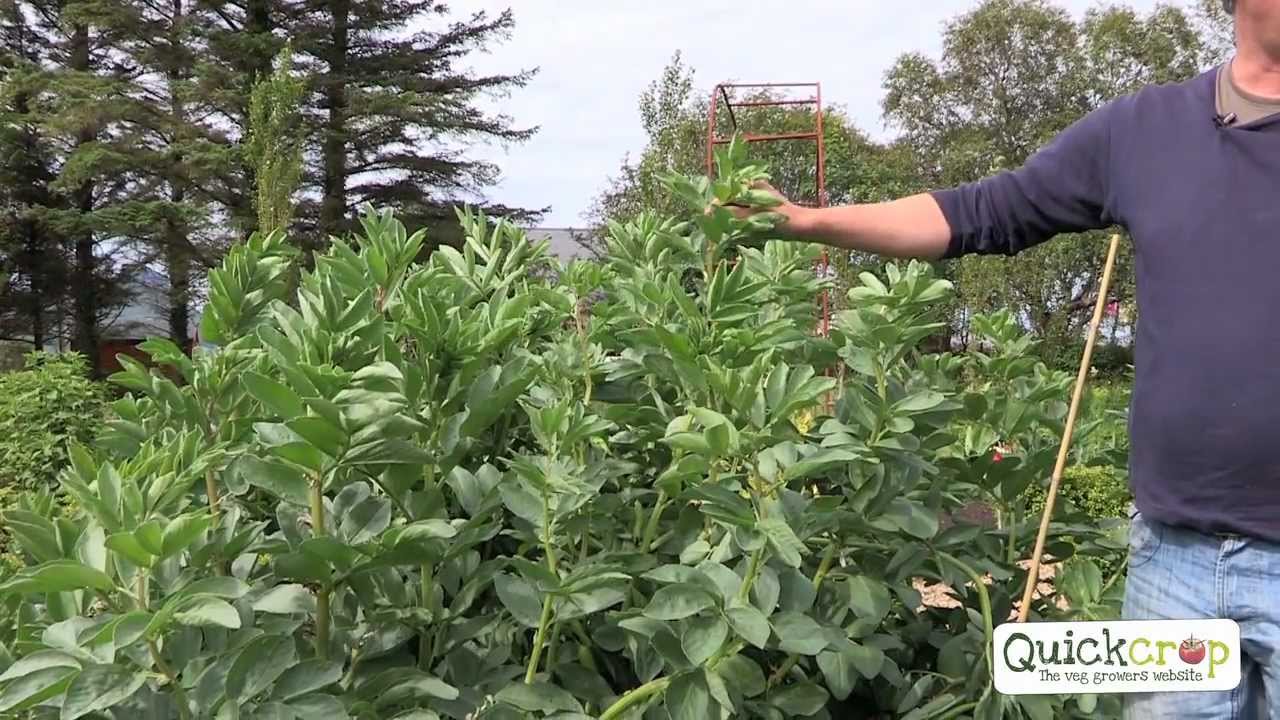The image depicts a daytime outdoor scene set in a natural environment, showcasing a garden abundant with tall, leafy plants that resemble fava beans. These plants, positioned in the foreground, are almost as tall as a man standing to the right, who wears a gray long-sleeved shirt with the sleeves rolled up and blue denim jeans. Visible to the left are a mix of dark green pine trees and lighter-hued trees under a somewhat cloudy, gray sky. In the middle right of the image, there is text within a light-colored rectangular insignia that reads "Quick Crop: The Veg Grower's Website," with the 'O' in "crop" creatively depicted as a tomato. An orange structure can also be glimpsed in the background, adding an additional layer of detail to the natural setting. The overall color palette includes various shades of green, forest green, white, black, faded blue-green, and tan beige.